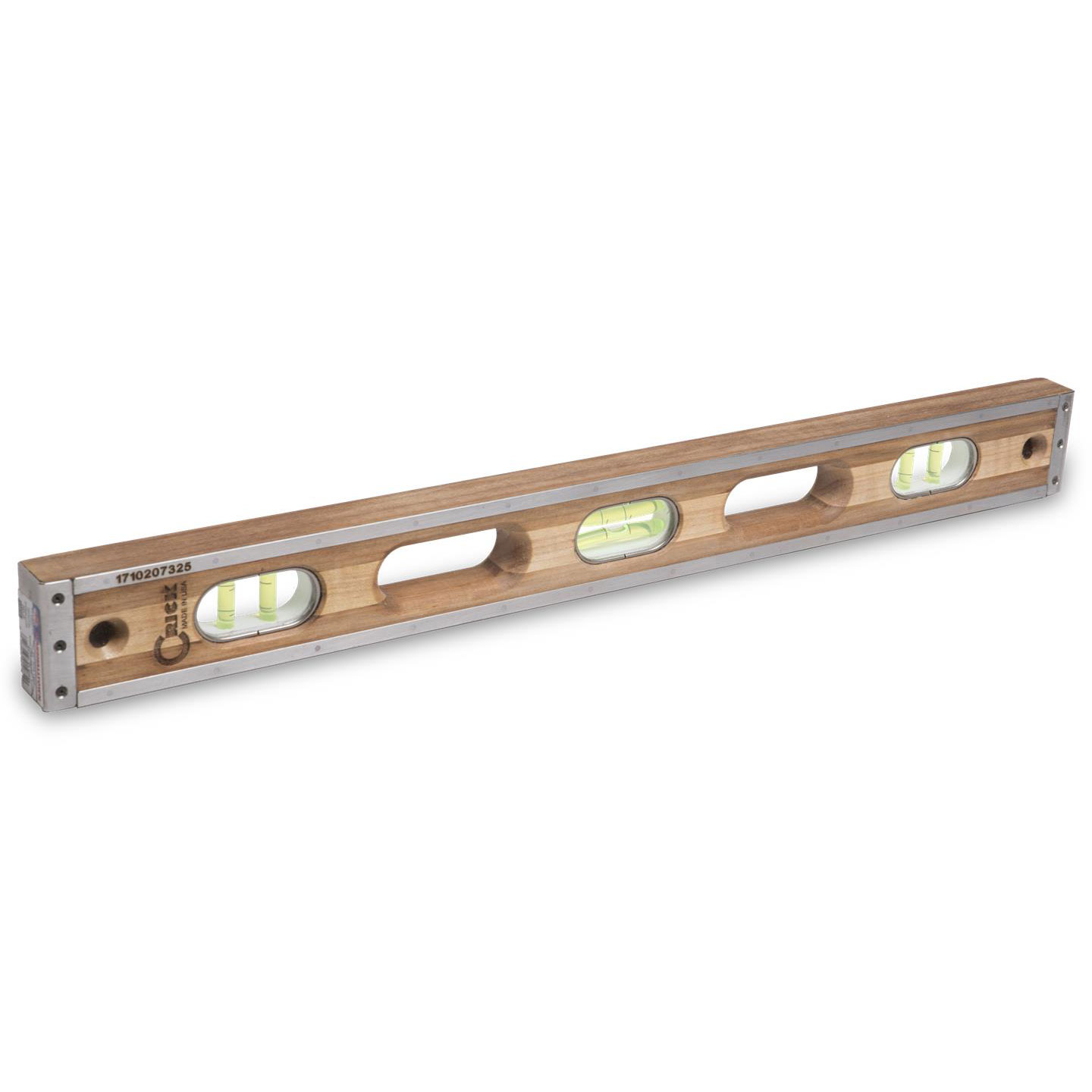This photograph, set against a plain white background, showcases a meticulous close-up of a precision tool: a wooden level. This level, featuring a light wood grain pattern, is accentuated with chrome or silver-colored metal pieces along its front, sides, and ends, adding both durability and a touch of sleekness. On the metal section at the upper left corner, the numbers "1710, 207, 325" are clearly inscribed. Below this on the wooden part is the brand name "Crick," indicating that it is made in the USA. 

The level contains three distinct cut-out oval sections housing liquid-filled vials that act as indicators. These vials are strategically placed; two are positioned vertically at each end to measure vertical alignment, while one sits horizontally in the middle to check horizontal alignment. Each vial contains green liquid with a small bubble, which settles between two black lines to indicate if the surface is level. On both sides of the horizontal vial, there are ergonomic handgrips for ease of use. Additionally, the metal pieces on each end feature three decorative circles, adding to the tool's aesthetic without compromising functionality.